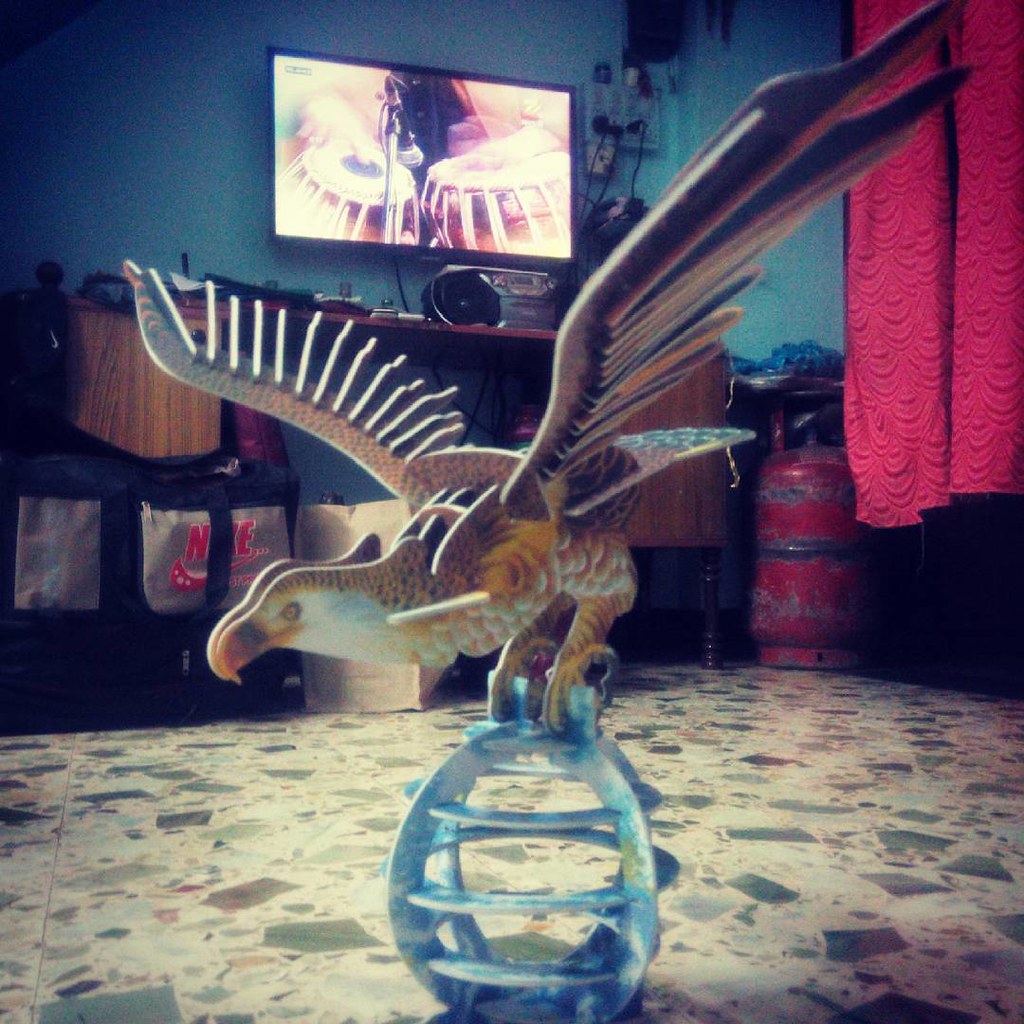This indoor photograph depicts a 3D eagle puzzle, meticulously constructed from cardboard or painted wood, perched authoritatively atop a light-turquoise globe. The eagle, featuring brown wings, a white underside, and a distinctive hooked yellow beak, rests its detailed talons on the blue orb. This scene unfolds against an off-white, somewhat grainy floor, accented with scattered patches of green, brown, and red that resemble a nougat slice with dried fruit.

In the background, a blue wall provides a stark contrast to the image's finer details. A flat-screen television, mounted to the blue wall, shows what appears to be a fragmented or spiky image, hinting at an adventurous scene possibly from Game of Thrones. Adjacent to the television, on the right side, red curtains hang gracefully, adding a bold splash of color to the setting. The environment is further complemented by a wooden desk beneath the TV, adorned with various items including what looks like a CD player and a basket emblazoned with the Nike logo. The entire scene is subtly illuminated, capturing the intricacies of the eagle and the ambiance of the room, despite the photograph's slightly dark and grainy quality indicative of an older camera.